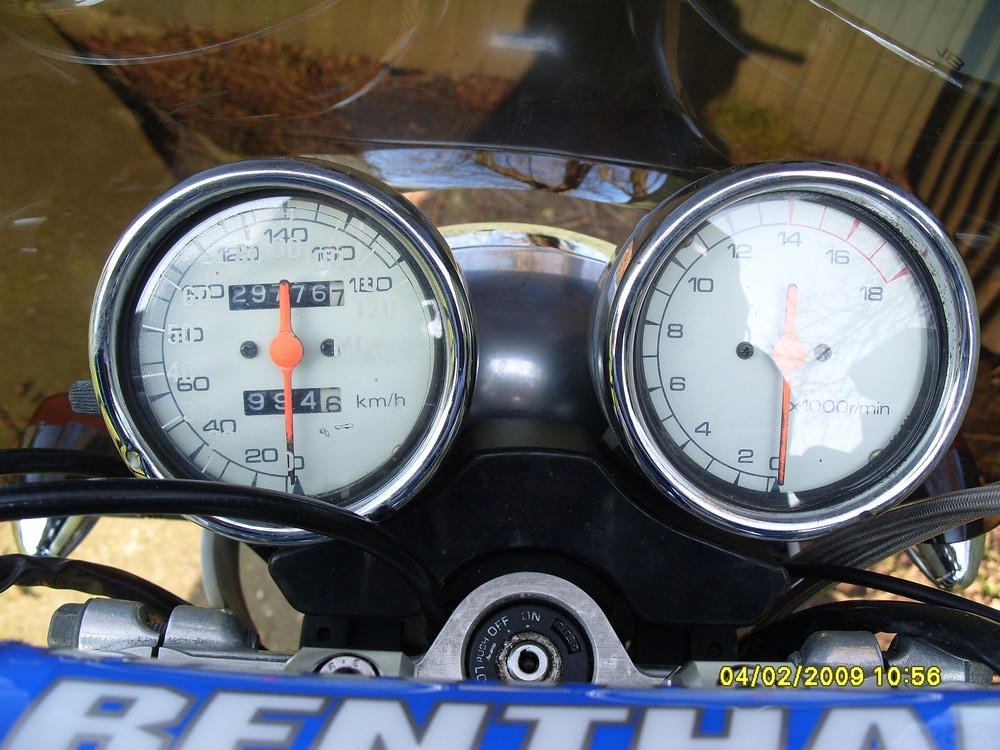A close-up photograph of a motorcycle dashboard showcases its intricately detailed controls. Dominating the view are two large, round dials, both encircled with gleaming chrome rims and featuring white faces. 

The dial on the left is a speedometer, marked prominently in kilometers per hour (km/h). Its orange needle currently rests at 0 but can move up to a maximum of 180 km/h. 

To the right is the tachometer, designed similarly with a chrome rim and white face but with a red needle. This dial measures engine speed in revolutions per minute (RPM), with a range from 0 to 18, representing 1000 RPM intervals. 

Below these meters, the black surface of the motorcycle's front panel is visible, housing an ignition switch identifiable by an 'off/on' marking. Wiring is also somewhat visible, extending from this area. Enhancing the dashboard's functionality, a transparent plastic shield is positioned above the two dials, likely serving as a protective cover.